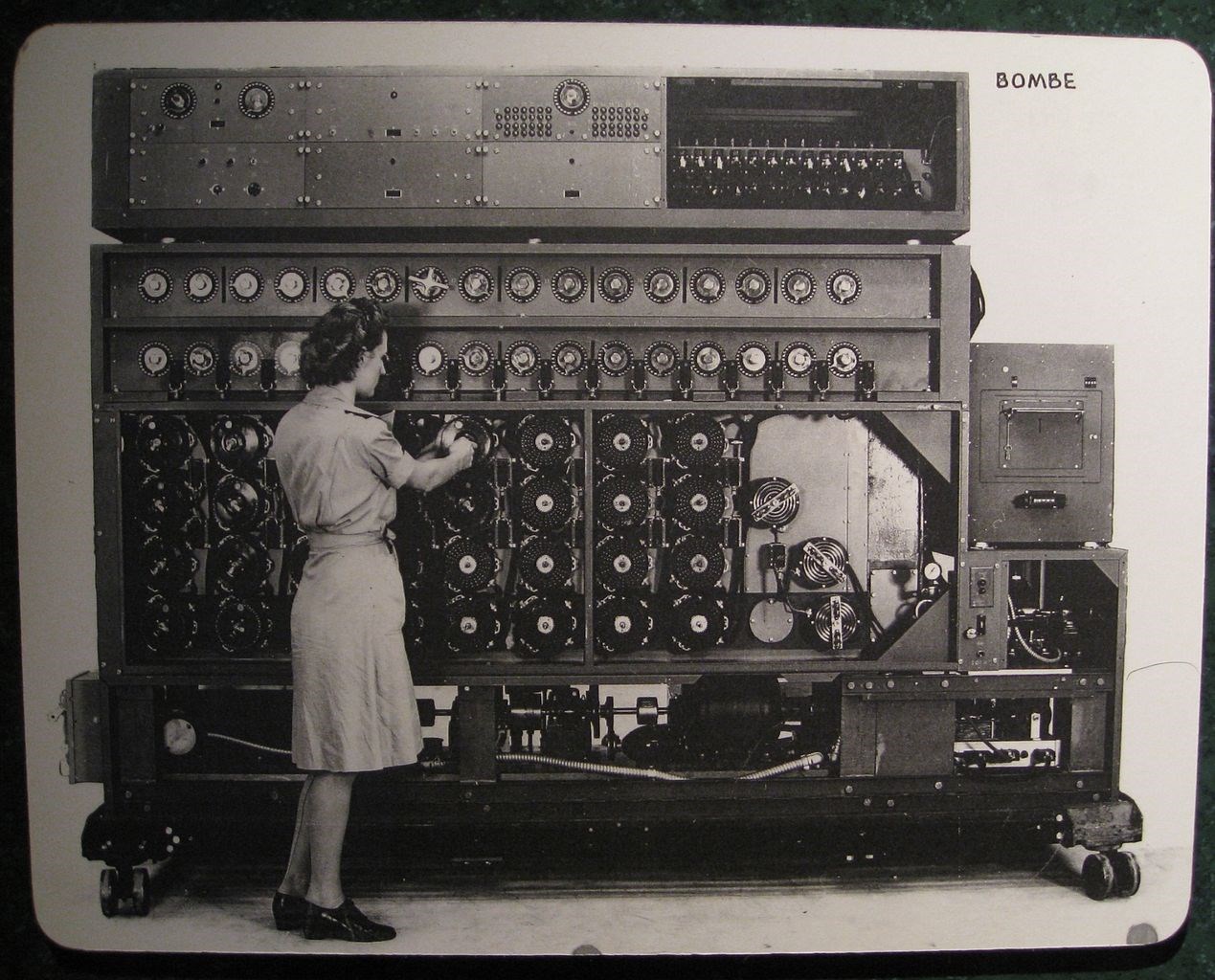In this black and white photograph, a woman dressed in a light gray dress tied at the waist with a collar, and black, shiny era-specific shoes, stands in front of a massive, pre-1950s machine labeled "BOMBE" in the top right corner. The woman appears focused as she manipulates one of the circular discs on the machine. The machine itself is an imposing, intricate device, nearly twice the height of the woman, mounted on wheels for mobility. Its complex structure includes columns of larger discs where the woman is working, surrounded by smaller discs above, and extensive metal panels filled with switches, dials, and gauges at the top. The bottom part of the machine exposes various wires and rods, hinting at its sophisticated electrical operation. The dark machine contrasts starkly against the white background, highlighting its formidable and enigmatic presence.